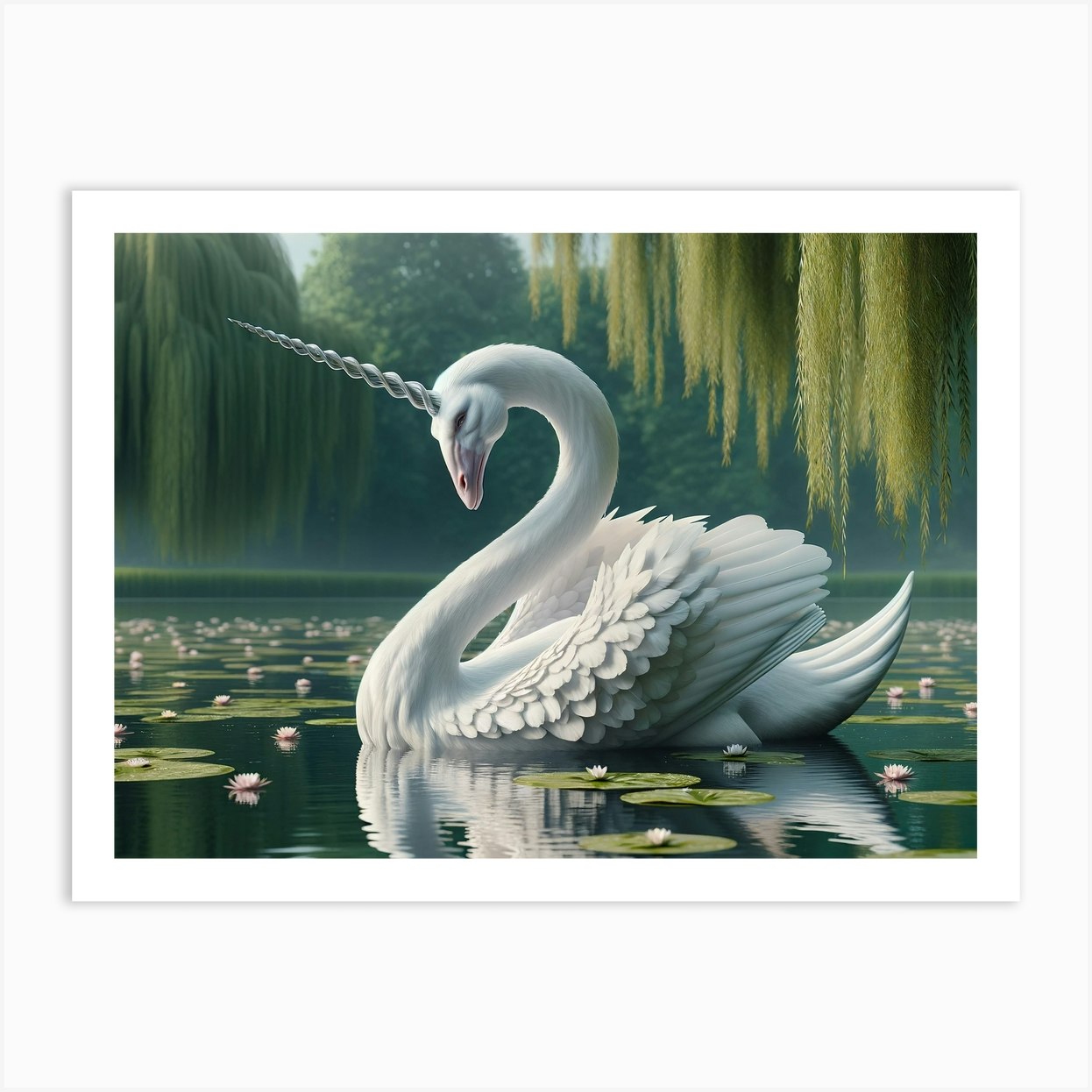This image is a detailed painting of a fantastical creature dubbed a "swanicorn" (trademark pending), primarily focused on a striking, surreal white swan with unicorn-like features. The centerpiece of the artwork is the extraordinary swan swimming gracefully in a greenish pond adorned with green lily pads and scattered white and pink flowers. 

The swan's body is entirely white except for a light pink area around its beak, and it has a large, spiral silver horn about four inches long emerging from the top of its head, adding a mystical element to its appearance. The swan's neck creates a backward "S" shape, curving elegantly up and then down, before gracefully sweeping to the right. Its head is tilted leftward with an intense, almost diabolical expression, giving the creature a unique, almost otherworldly demeanor.

The swan’s wings are large, feathered, and slightly ruffled, positioned tensely as if in mid-motion, which, along with its aggressive facial features, adds to its surreal and slightly ominous presence. Its full, white tail extends to the right, contributing to the dynamic composition of the scene. 

The serene pond reflects the swan's image clearly, only slightly disturbed by its movement. The background is rich with greenery, featuring willow-like trees with long, hanging leaves and other lush foliage lining the shoreline. Through the tops of these trees, patches of blue sky are visible, adding depth and tranquility to the serene landscape. This blend of peaceful scenery with the swan's intense demeanor creates a captivating and thought-provoking piece of art.